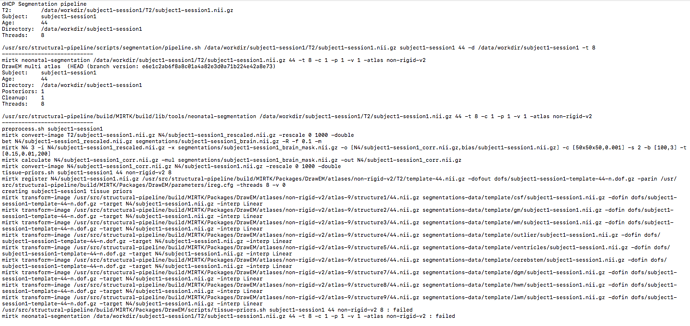The image showcases a document with a white background and predominantly black text, with extensive content that appears to involve programming or technical documentation. The document is divided into multiple sections. 

The first section is titled "DHCP Segmentation Pipeline," and it includes a code snippet: "T2 = data worker" followed by the directory address. It also mentions a subject with additional details such as "subject session age 44" and another directory address, with threads set to zero.

The second section lists a directory containing detailed information. Notably, it specifies "subject" with the values "subject one, session one, age 44." This section also includes directories labeled "Posteriors one," "Cleanup one," and "Thread zero."

The final section is a dense block of text, featuring an extensive list of directory folders and their respective addresses. This section spans over 20 lines and heavily suggests a context related to coding or data management.

Overall, the document appears to be a detailed technical guide or configuration file related to a data processing pipeline.